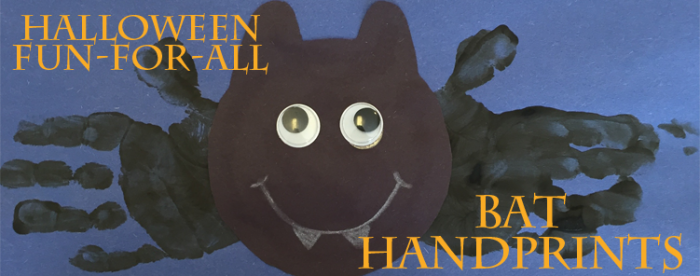The image is a horizontally aligned, wide rectangular picture set against a dark blue background, likely construction paper. It features an artistic depiction of a bat creature in the center. The bat's face is circular with pointy ears made out of felt, and it has large googly eyes with black and gold centers that are glued onto the face. A curved, gray smile with two small, triangular vampire teeth is drawn underneath the eyes. Flanking the face are black handprints, made to look like the bat's wings, as if someone dipped their hands in black paint and pressed them onto the paper. In the top left corner, yellow all-caps text reads "HALLOWEEN FUN FOR ALL," and in the bottom right corner, orange all-caps text stacked vertically reads "BAT HANDPRINTS." The blue background and the playful elements suggest a fun, Halloween-themed arts and crafts project.